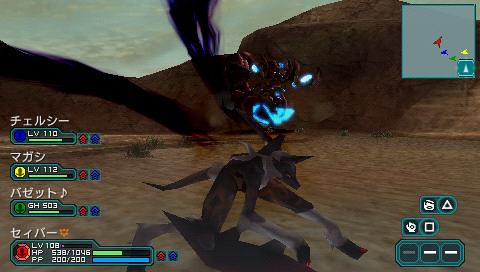The image depicts a video game screen brimming with various elements and details. In the top-right corner, there is a gray box functioning as a map, adorned with colorful arrow-tip shapes in yellow, green, blue, and red. The backdrop of the game showcases brown mountainous or hilly terrain under a blue-green sky partially obscured by gray clouds. On the left side of the screen, three identical rectangular shapes followed by two square shapes come into view, each labeled with either Chinese or Japanese characters. These elements are accompanied by levels marked as 110, 113, and 112, along with the code GH503.

Below this sequence, a larger instance of the same shape displays additional information: a level of 108, health points (HP) reading 538 out of 1046, and power points (PP) at a full 200 out of 200. Dominating the center part of the screen is a dog-like creature, easily identifiable by its gray and darker patches of fur. In the background, there is something pinkish-reddish with blue accents that adds an intriguing splash of color to the scene.